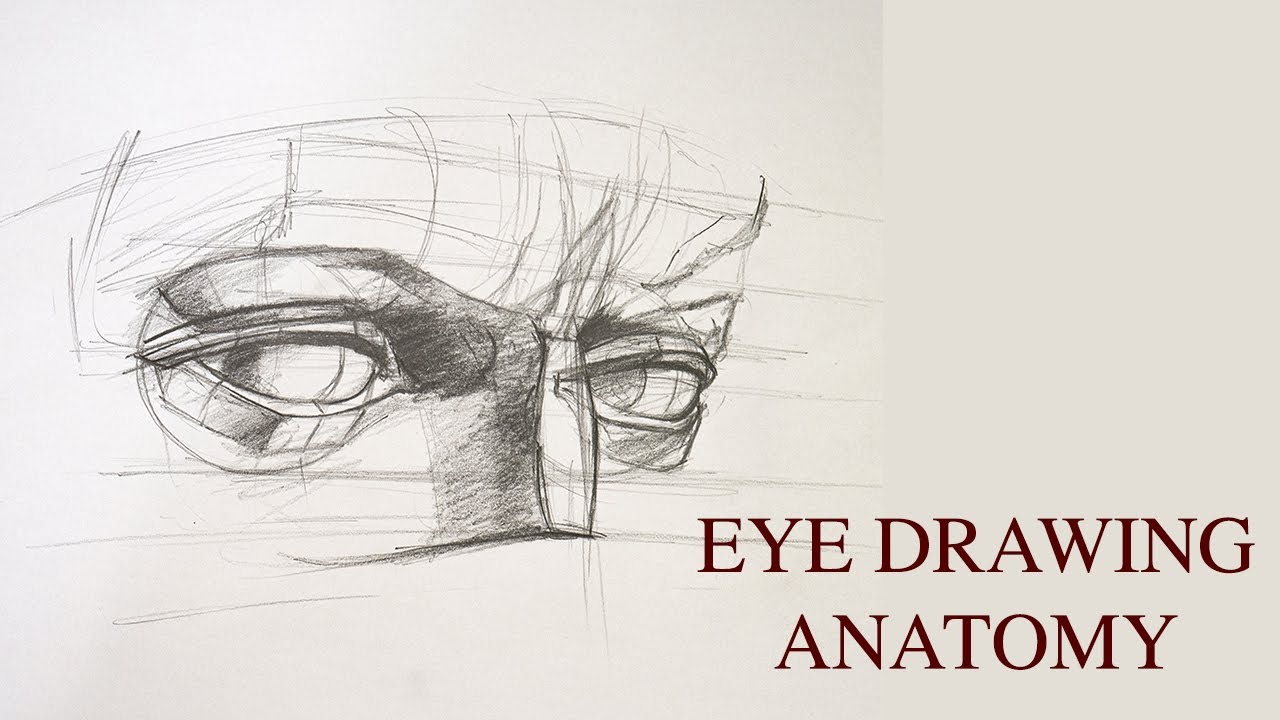The image features a partial pencil sketch of a human face set against an off-white or cream-colored background. The focus of the drawing is on the eyes and the upper bridge of the nose, which taper off into unfinished lines extending to about half of the forehead and nose. The sketch uses darker shading near the nose, which gradually lightens around the eyes, creating a focused intensity as the eyes give a sideward gaze. In the bottom right corner, text in dark red letters reads "Eye Drawing Anatomy." This emphasizes the instructional or illustrative nature of the artwork.